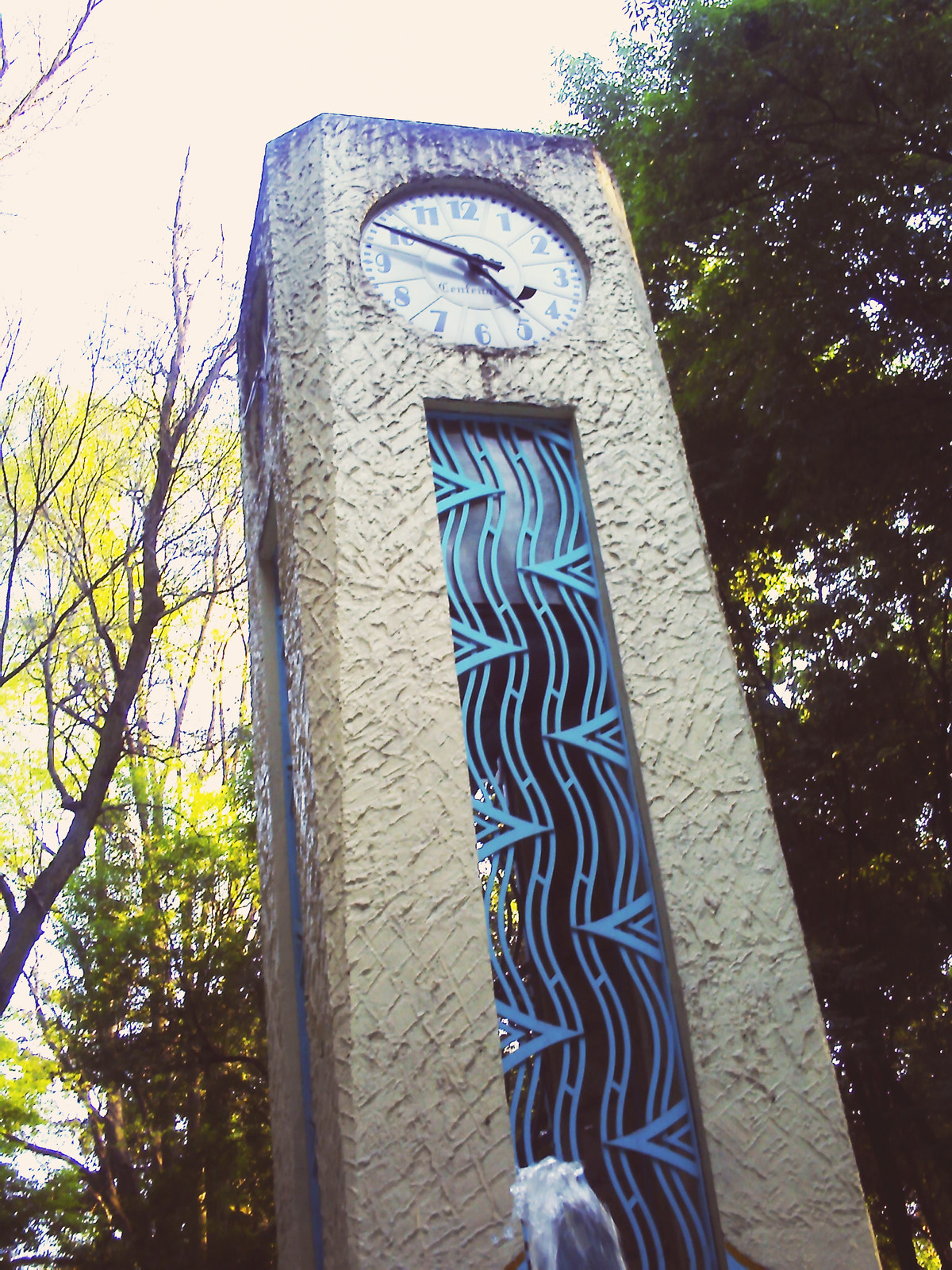This color photograph, taken outdoors during the day, prominently features a large rectangular stone clock tower. The tower has a textured tan surface punctuated with black spots of discoloration, indicating potential water damage, particularly at the top. The clock face, located at the top of the structure, displays the time as a little bit over a quarter till five, with black hands and Arabic numerals bordered with thicker black lines and minute denotations in thin lines. The clock face itself might be silver or tan, obscured by the angle and lighting, and features a small cursive label in the center. 

Beneath the clock face, the tower boasts an intricate inlay of blue glass, framed by wavy cyan blue lines separated by vertical sections and flanked by triangles. The background reveals a varied landscape with tall, dark green trees to the right and shorter trees with lighter-colored leaves on the left. The sky in the top left corner appears bright, contrasting with the grayish hue dominating the rest of the sky. Near the base of the tower, there seems to be a fountain shooting up water, adding a dynamic element to this sculptural centerpiece.